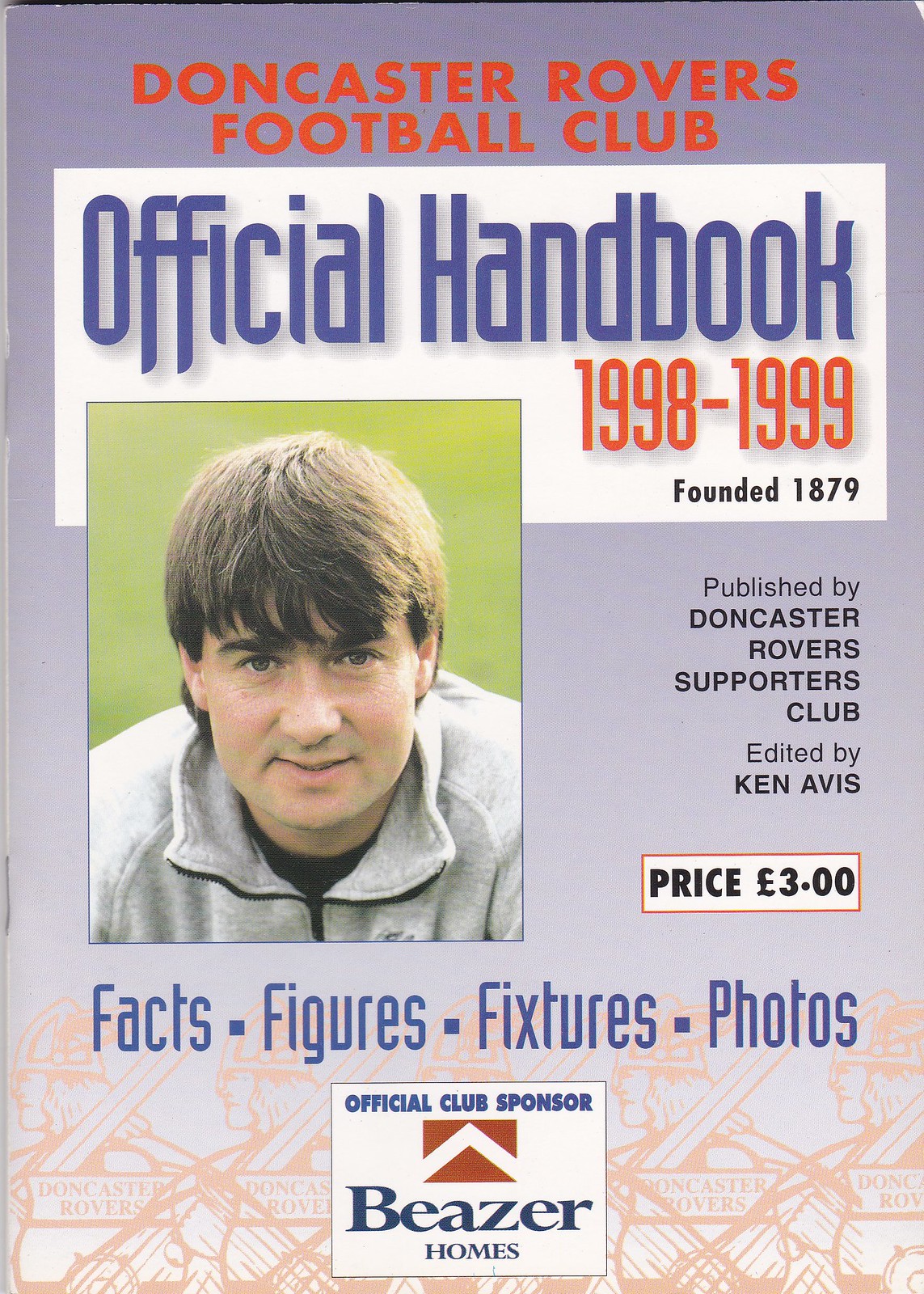The cover of the official handbook for Doncaster Rovers Football Club for the years 1998-1999 is prominently displayed. The handbook is titled in dark blue letters that read "Official Handbook 1998-1999" on a white background. Above this title, on a dark blue band, the words "Doncaster Rovers Football Club" are written in orange, with the club's founding year, 1879, noted in black below it. A photograph of a cheerful young man with brown hair and bangs, wearing a light gray fleece jacket, is centered on the cover. The image has a green background. To the right of this photo, the price of the handbook, £3, is listed in black lettering. Additional text includes "Published by Doncaster Rovers Supporters Club" and "Edited by Ken Avis." The cover also highlights that it contains facts, figures, fixtures, and photos, with these words written in blue letters. The official club sponsor, Beezer Homes, is acknowledged with blue lettering on an advertisement panel. The entire design incorporates a color scheme of maroon, blue, and white on a gray background. At the bottom, images of a Viking holding a sword and wearing a helmet are depicted with the words "Doncaster Rovers" in the center.